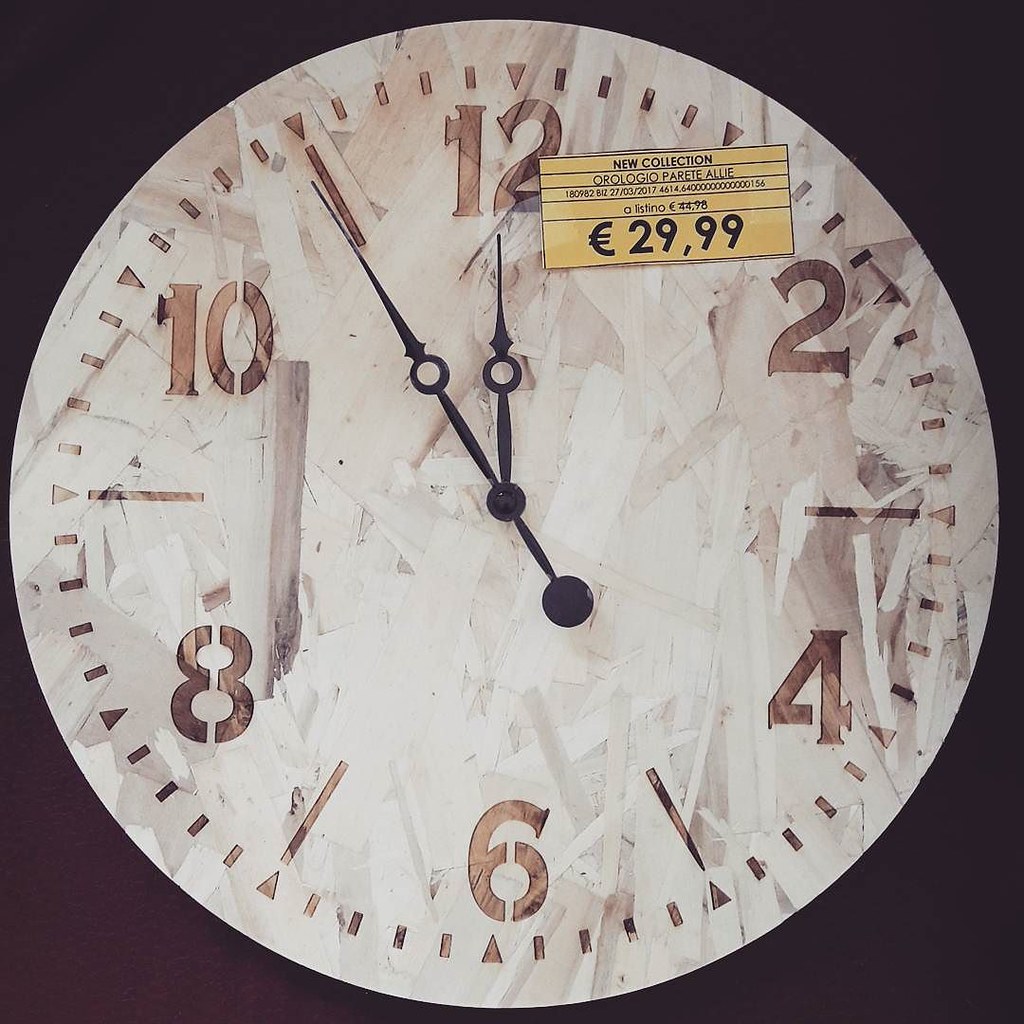This image features a square-shaped clock prominently displayed against a almost-black background with subtle reddish-brown undertones. The antique-style clock face dominates the composition and showcases faded stencil-style numbers for the hours of 12, 2, 4, 6, 8, and 10, with simple markers for the intervening odd hours. The clock is equipped with elegant cast iron hour and minute hands, and a distinctive bulb-tipped second hand sweeping the face. A tag attached to the clock reads "New Collection," or "Logio Parete Alia," priced at €29.99, indicating it's part of a European sale. The clock's overall aesthetic is both artistic and vintage, evoking a timeless, classic appeal.